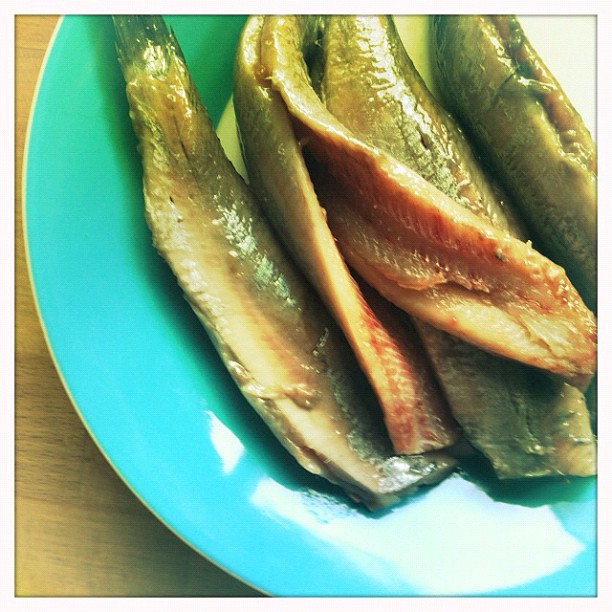The image captures a close-up view of four headless sardines arranged on a round plate with a turquoise blue border and a white center. One of the sardines is cut open, revealing its pinkish internal meat, while the outer skin of all the fish displays a brownish-grey hue. The fish, with their fins still intact, are positioned on a wooden table that features a light yellowish tone with dark designs. Sunlight from the upper right corner of the image casts a warm, yellowed tint over the scene, adding a rustic feel to the composition.